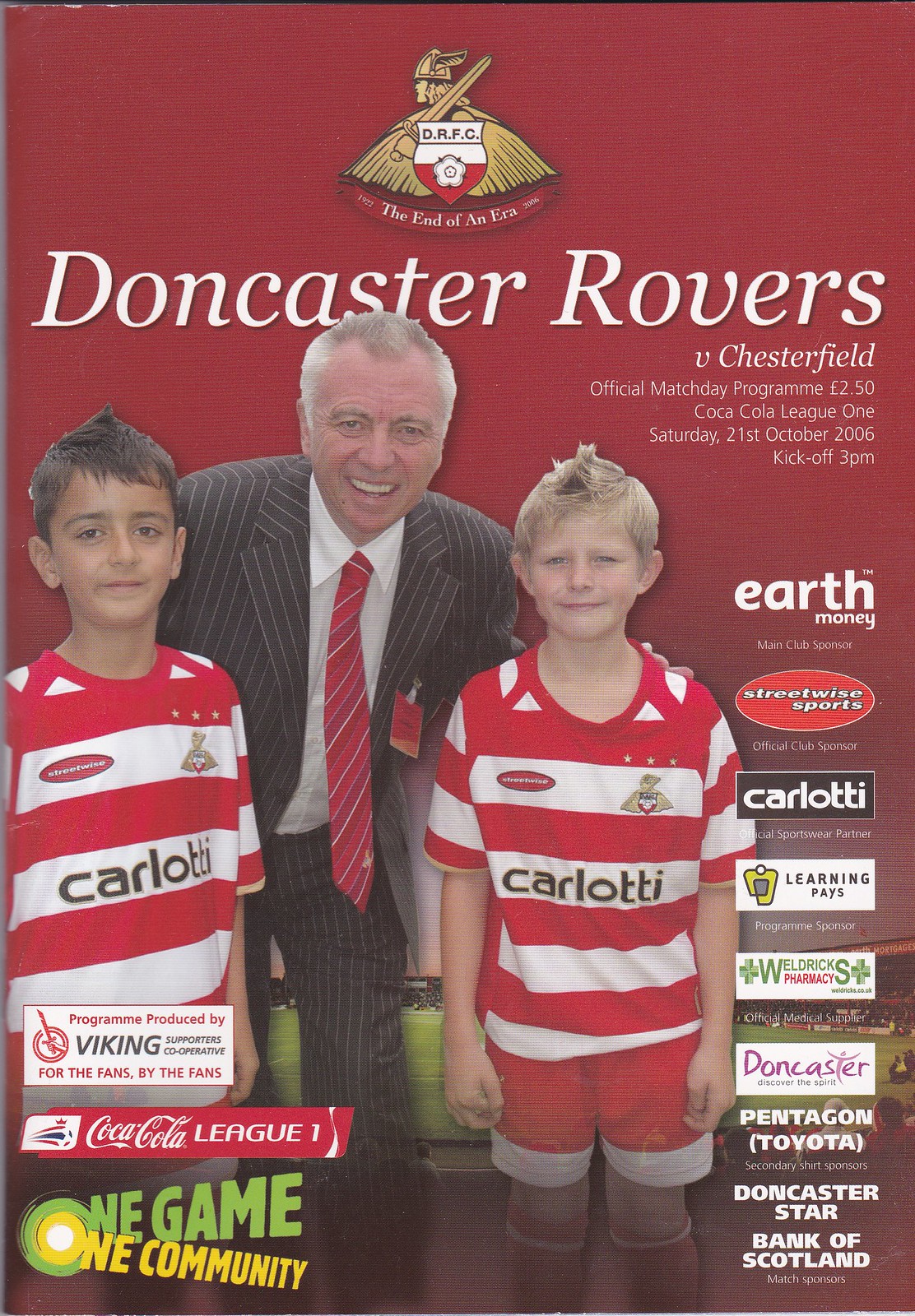This is the official matchday program cover for the Doncaster Rovers Football Club, highlighting their game against Chesterfield in the Coca-Cola League One on Saturday, October 21, 2006, with a kickoff at 3 p.m. The cover, predominantly red, features a striking image of an older Caucasian man donned in a gray suit with a red tie, standing behind two children who are dressed in matching red and white horizontally-striped jerseys with red shorts and white accents. One child has dark hair and the other is blonde. The title "Doncaster Rovers vs. Chesterfield" appears at the top, beneath the club logo "DRFC, 1922, the end of an era, 2006". The sponsors, including Earth Money, Streetwise Sports, Carlotti, Learning Pays, Weldrick's Pharmacy, Doncaster, Pentagon Toyota, Doncaster Star, Bank of Scotland, and "One Can Be One Game," are listed alongside the right. The program, produced by Viking Supporters Cooperative, carries the motto "for the fans by the fans," emphasizing the community spirit of the event. The overall composition, incorporating colors like burgundy, red, yellow, green, black, white, gray, purple, and beige, positions the trio centrally, capturing their image from shin-level upwards.